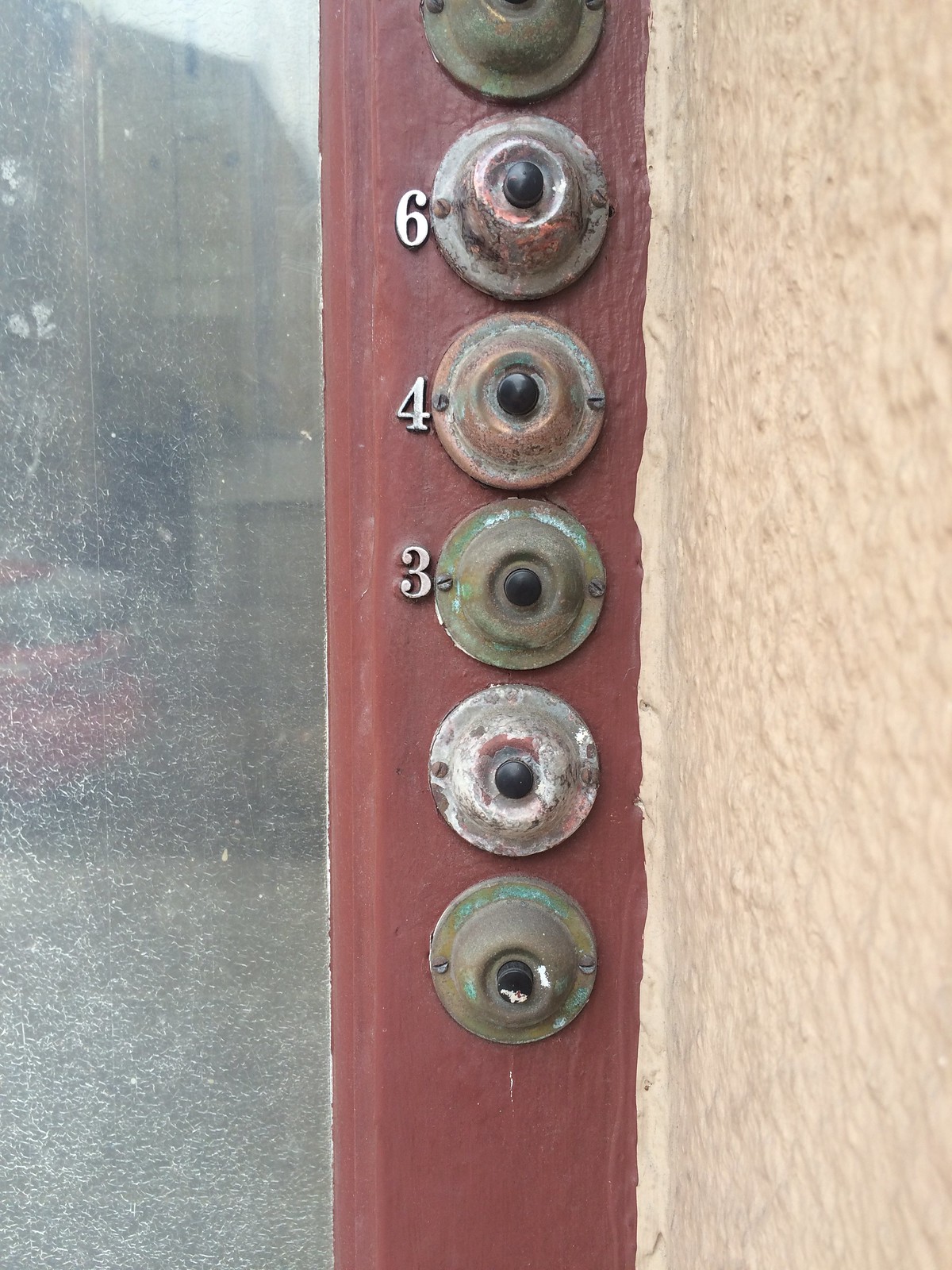This close-up photograph captures the side of an apartment building's see-through door, emphasizing a reddish-brown painted rectangular doorframe. The frame features six stacked, antiquated metal doorbells with black press buttons, each showing signs of age and wear. The doorbells vary in color from patinated brown to light tan, suggesting they might have been white initially. Three of these doorbells are accompanied by numbers on the left: a "6" next to the fifth bell from the bottom, a "4" beside the fourth, and a "3" near the third. Adjacent to the right of the doorframe is an orange-colored stucco wall forming a corner, highlighting the aged texture and color transition of the building's exterior. To the left, a glass pane of the door reveals a dusty windowsill inside, though details remain indistinct.